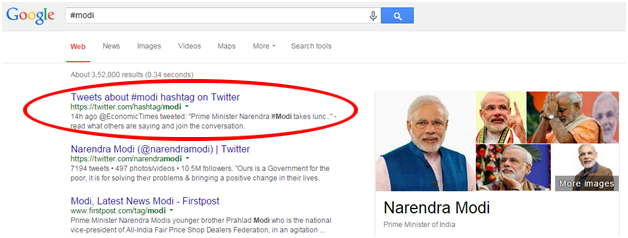The image depicts the top segment of a Google search results page. Against a light gray border at the top, the distinctively colorful Google logo comprising shades of blue, red, yellow, green, and more red is prominently positioned to the far left. A search box, located centrally, displays the typed query "#MODI" in black print. Adjacent to the search bar are a blue "Search" button and a gray microphone icon for voice searches.

Directly underneath the search bar, the webpage background transitions to white. Several navigation tabs—Web, News, Images, Videos, Maps, and More—are conspicuously listed at the top. An icon to the right of these tabs provides additional options when clicked, labeled "Search tools." Below these tabs, the search result count is displayed, indicating approximately 3,052,000 results retrieved in 0.34 seconds.

Highlighted prominently, a red marker has circled the top result which states "Tweets about #MODI." This indicates user-generated content related to the hashtag #MODI on Twitter. Accompanying this result is the URL linking directly to the hashtag page on Twitter. Further down, additional links appear, including one directing to the official Narendra Modi Twitter handle (@narendramodi), and another pointing to "MODI latest news," within the website "Firstpost."

On the right side of the page, a visual panel showcases several images of an older gentleman with tanned skin and light-colored hair and beard; the person is identified as Narendra Modi.